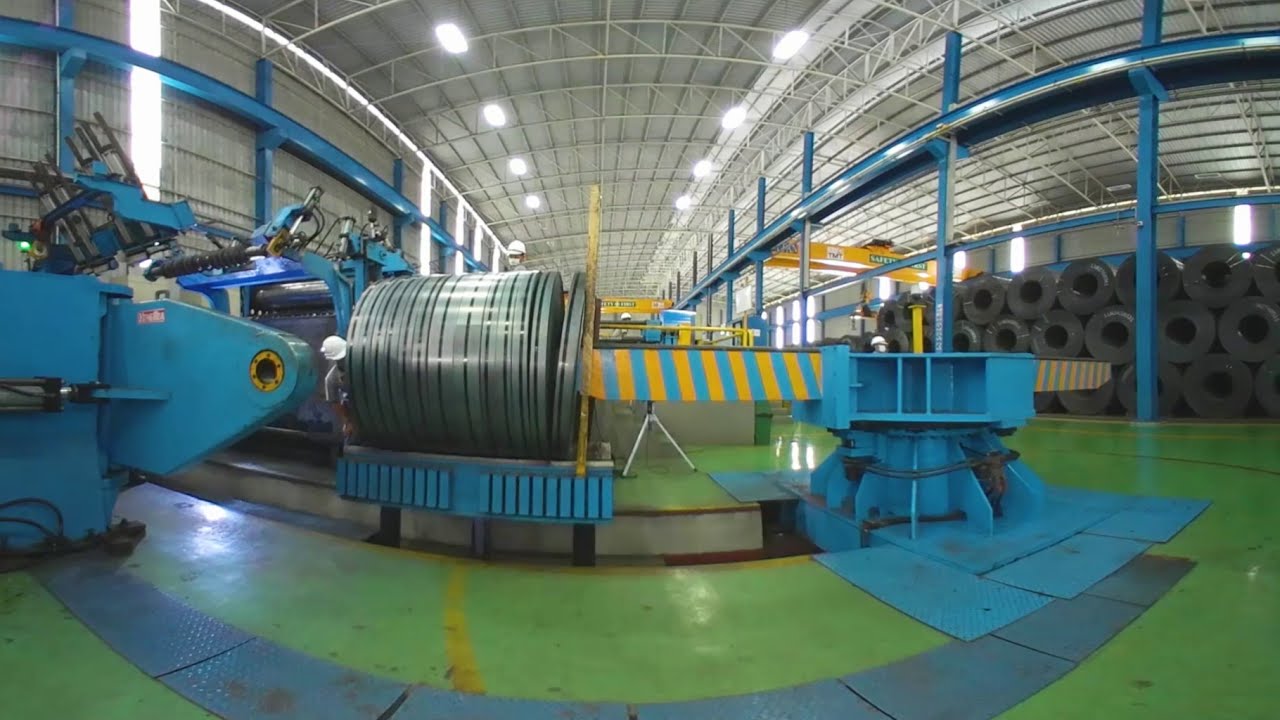The photograph captures an expansive indoor setting within a factory, characterized by its corrugated metal walls and ceiling supported by both blue and silver beams. Rectangular in shape and devoid of any border, the image is illuminated by bright white lights hanging from the high ceiling. The factory floor is primarily moss green with areas featuring blue metal panels equipped with a textured surface for light traction. Dominating the scene is blue machinery accented with white stripes, alongside large, stacked gray discs that resemble big silver rings or tire-like objects. On the left of these discs, a man wearing a white hard hat is visible, while another similarly helmeted individual peeks over the top of the stacks. Additional caution areas are marked by yellow and blue stripes, and more rolls or products can be seen stacked in the distance. The overall ambience of the image is marked by a persistent blue hue, juxtaposed against the green and yellow elements of the floor, giving the setting an old-fashioned yet industrial feel.